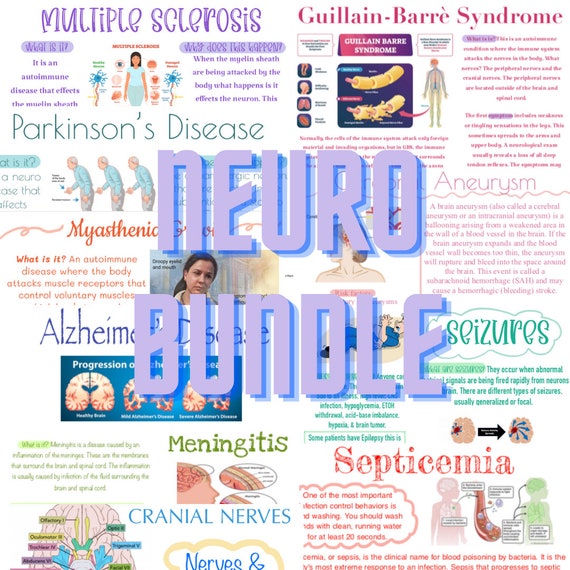The image is a detailed, color-coded infographic titled "Neural Bundle," prominently displaying information on various neurological disorders and diseases. Set against a background that transitions from white to gray-purple, the infographic is laid out in an organized fashion resembling a polished collage. In the upper left corner, the section on multiple sclerosis is highlighted in purple, with detailed text and a corresponding illustration. To the right, there's a part dedicated to Guillain-Barré syndrome, followed below by a section on Parkinson's disease, each accompanied by descriptive text and relevant images. Additional sections include Alzheimer's, showcasing the progression of brain tissue, and an overview of meningitis, cranial nerves, seizures, an aneurysm, and septicemia. Each section uses various colors like purple, blue, orange, and green to differentiate the conditions, making the infographic visually engaging and informative. This poster, which could be seen in a doctor's office or a school, offers crucial information on brain health and neurological conditions, making it an invaluable educational tool.